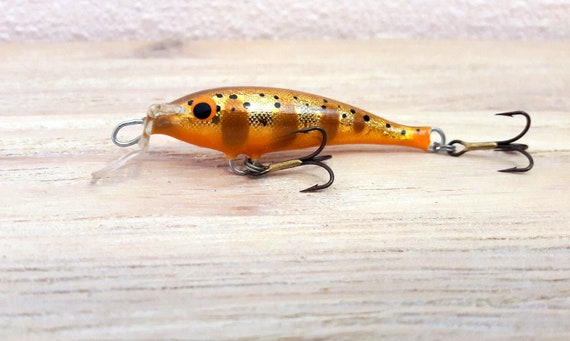This horizontally oriented photograph captures a detailed close-up of a specialized fishing lure resting on a white, horizontally striated wooden surface. At the top of the image, the texture changes to a rougher, styrofoam-like material. The lure, designed to mimic a small fish or minnow, features a yellow body adorned with black spots and brown vertical stripes. It measures approximately 1.5 to 2 inches in length. A large, round black eye is positioned near a small steel loop protruding from its mouth, indicating how it would attach to a fishing line. The lure is equipped with two black, multi-pronged treble hooks; one hangs from the midsection, and the other is affixed at the tail. This bait's design and coloration suggest it is intended to attract fish, although the specific type it is meant to lure remains unclear.